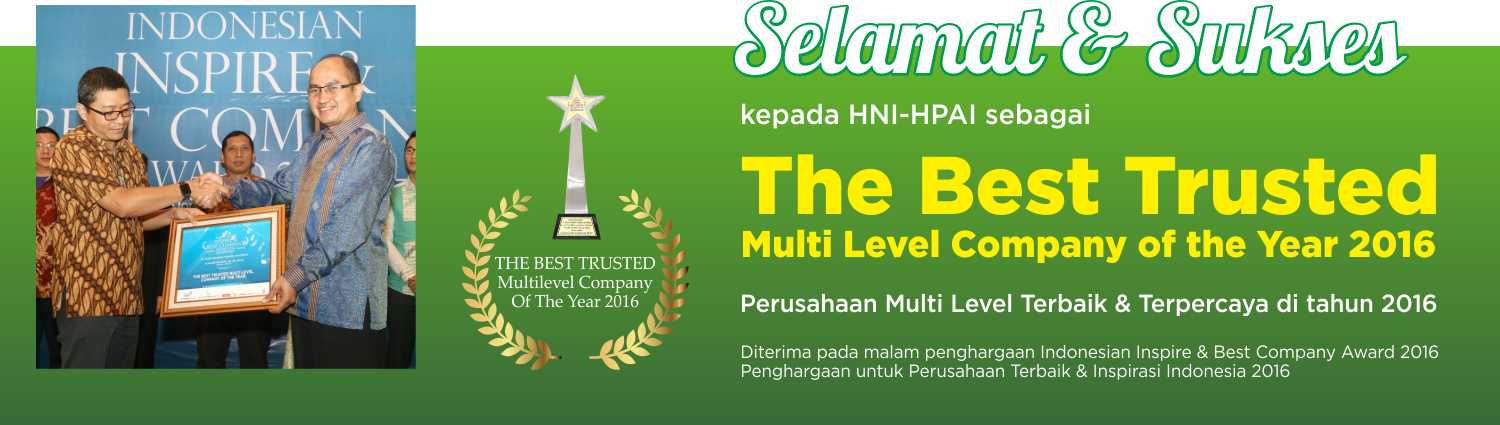The advertisement is a horizontal rectangle with a solid green background. On the left side of the banner, there is a square image featuring several people, with three men prominently in the center and one person in the background on each side. The two central men are shaking hands and holding a blue and white plaque, with one man in a brown patterned top and dark pants, and the other in a blue long-sleeved shirt and dark pants. Both are wearing glasses. Above them, large white, all-caps text partially obscured by their heads reads "Indonesia, Inspire, [obscured]". 

To the right of this image is a trophy-like logo, featuring a star on top and two gold half-circles surrounding it. Below the logo, white print proclaims, "The Best Trusted Multi-Level Company of the Year 2016."

Further to the right, against the green background, large white text says "SELAMAT" and "SUKSES." Underneath that, in smaller white letters, it reads "Kepada HNI-HPAI Sebagai." In the middle, in bold yellow letters, is the declaration, "The Best Trusted Multi-Level Company of the Year 2016." Below this in smaller white text are additional details primarily in another language, indicating further accolades and recognition.